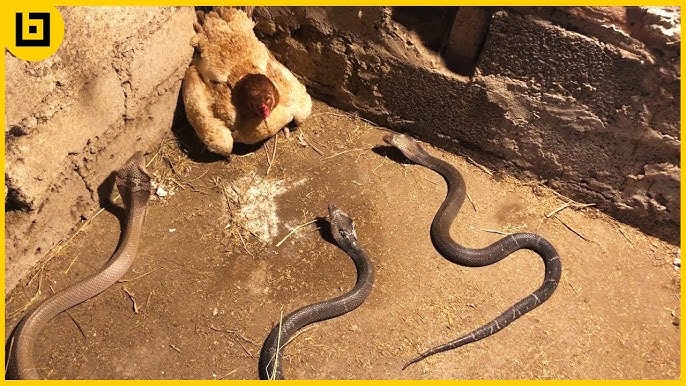In the image, a terrified chicken with a white body, brown head, and red beak is cornered at the intersection of two rough, uneven stone walls. The setting features compact, hard-packed dirt ground. Three cobras, each poised with their bodies partially lifted off the ground and tongues flicking, are closing in on the cowering chicken. The snakes, brown and sinister, exhibit an air of imminent threat, suggesting an impending attack on the trapped bird. Additionally, there is a symbol resembling the letter "B" in the upper left-hand corner of the image, outlined in yellow and black. The photograph captures a scene filled with tension and danger as the central focus remains on the menacing cobras and the helpless chicken within this confined space.